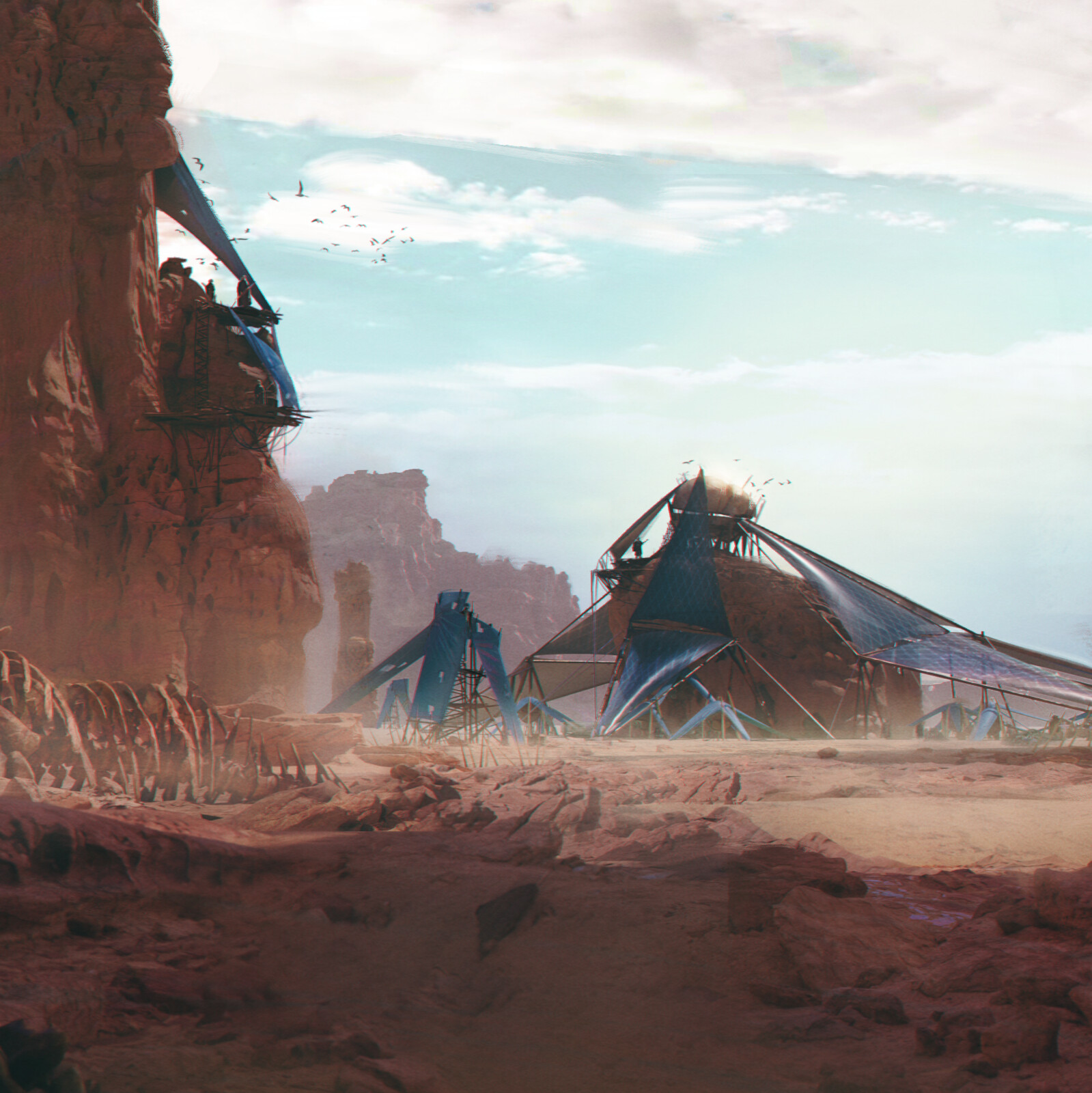A desolate, sandy desert landscape is dominated by a large, skeletal remains of a 20-foot-long creature, lying picked apart and weathered to the left side. The foreground consists of sand and pink-hued rocky ground, extending from left to right, where the skeleton rests. Rising from the middle left to the upper left of the image is a 25-foot-tall rock outcropping, adorned with blue tarps and material forming makeshift awnings and structures. These blue canopies, possibly once supported by thin poles, now appear to be collapsing or falling down. In the middle and right sections of the image, smaller rock formations cling to similar blue fabric, creating a stark contrast against the natural rocky environment. The backdrop reveals additional rocky terrains and an expansive sky filled with scattered white clouds. High above, towards the upper left, a distant group of birds navigates the serene light blue expanse.